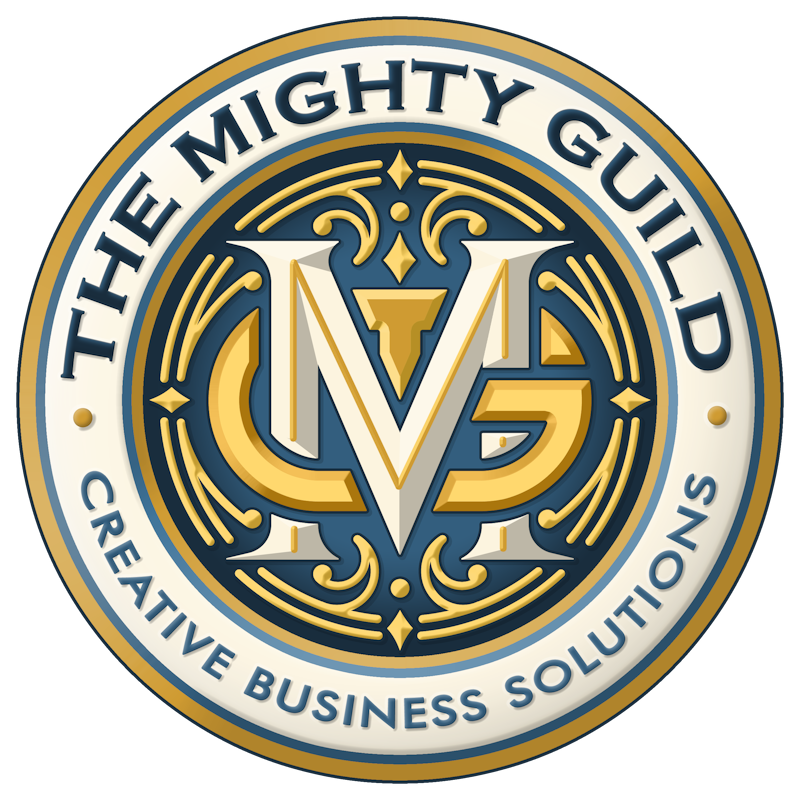The image is a detailed, close-up digital illustration of a guild logo presented in a circular format with a predominantly black background. The outermost edge of the circle features a light yellow or gold rim, followed by a narrow, light blue band. Inside this blue band is a thick white border that further encircles the logo. Text is displayed on this white border in dark blue, all capital letters; at the top it reads "The Mighty Guild," and at the bottom, it reads "Creative Business Solutions," both in curved text format. At the 3 and 9 o'clock positions on this white band, there are gold dots marking these points.

The central part of the logo is filled with elaborate decorative elements: a dark blue background with gold scrollwork and diamond shapes positioned at the 12, 3, 6, and 9 o'clock positions, creating a clock-like appearance. Dominating the center of this inner blue circle is a large capital "M" in white, which is thickly outlined in blue. This "M" intertwines with a smaller, light yellow "G," which is outlined in a darker gold. This combination of typography and graphic design elements delivers a sophisticated and professional logo emblem of "The Mighty Guild" and its associated entity "Creative Business Solutions."